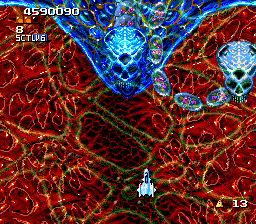In this screenshot from a video game, the upper left-hand corner displays a white score reading "4590090." Directly below this score is the number "8," followed by the alphanumeric sequence "5CTL6." A prominent graphic in the upper third of the image features a skull immersed in a blue, liquid-like texture, surrounded by liquid bubbles and vein-like structures that spread throughout the blue background. This blue imagery connects to another similar skull shape positioned to the right. The remainder of the background showcases an intricate web or labyrinth of red lines forming amorphous, closed loops, interspersed with larger closed loops of green, all set against a black backdrop. At the bottom of the screen is a small character in bright light blue, which has a distinguishable head and body but does not resemble a human. Lastly, the number "13" in white font is visible in the lower right corner of the image.